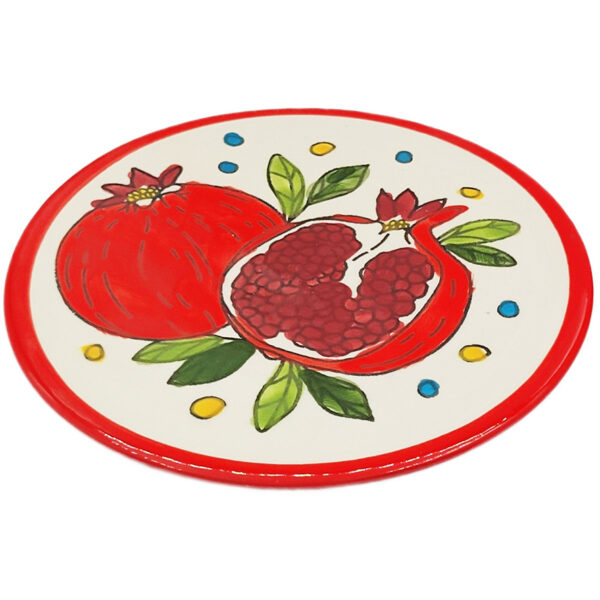This photograph showcases a circular ceramic trivet or coaster with a vibrant, artistic depiction of pomegranates. The white background is framed by a bold red rim that encircles the entire piece. On the left side, there is a whole pomegranate with a small star-shaped blossom scar facing up, its bright red and orange hues accented with subtle black streaks. Next to it, there is a pomegranate cut in half, revealing the intricate details of its interior. The inner flesh of the halved pomegranate is white, cradling clusters of deep burgundy seeds. The cut pomegranate is adorned with clusters of green leaves, four at the bottom and four at the top, varying from light to dark shades. Scattered across the composition are several blue and yellow circles, adding a whimsical decorative touch. The overall painting is vibrant and intricate, set on a stark white background that highlights the rich colors and detailed elements of the imagery.